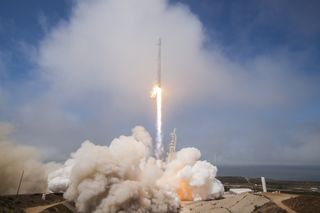In this vivid daytime image, we witness the powerful launch of a cylindrical rocket, centered in the frame and ascending towards an expansive blue sky. The bottom of the rocket emits a dramatic burst of orange fire, producing a thick plume of smoke that ranges from white to shades of brown and gray. Billows of white and gray smoke dominate the scene, with additional fluffy white clouds scattered throughout the sky. In the distance, the horizon reveals a glimpse of the ocean, adding depth to the background, while patches of green grass adorn the landscape below. The photograph captures the intense contrast between the rocket's bright flames and the serene blue expanse above, emphasizing the dynamic motion and energy of the launch.